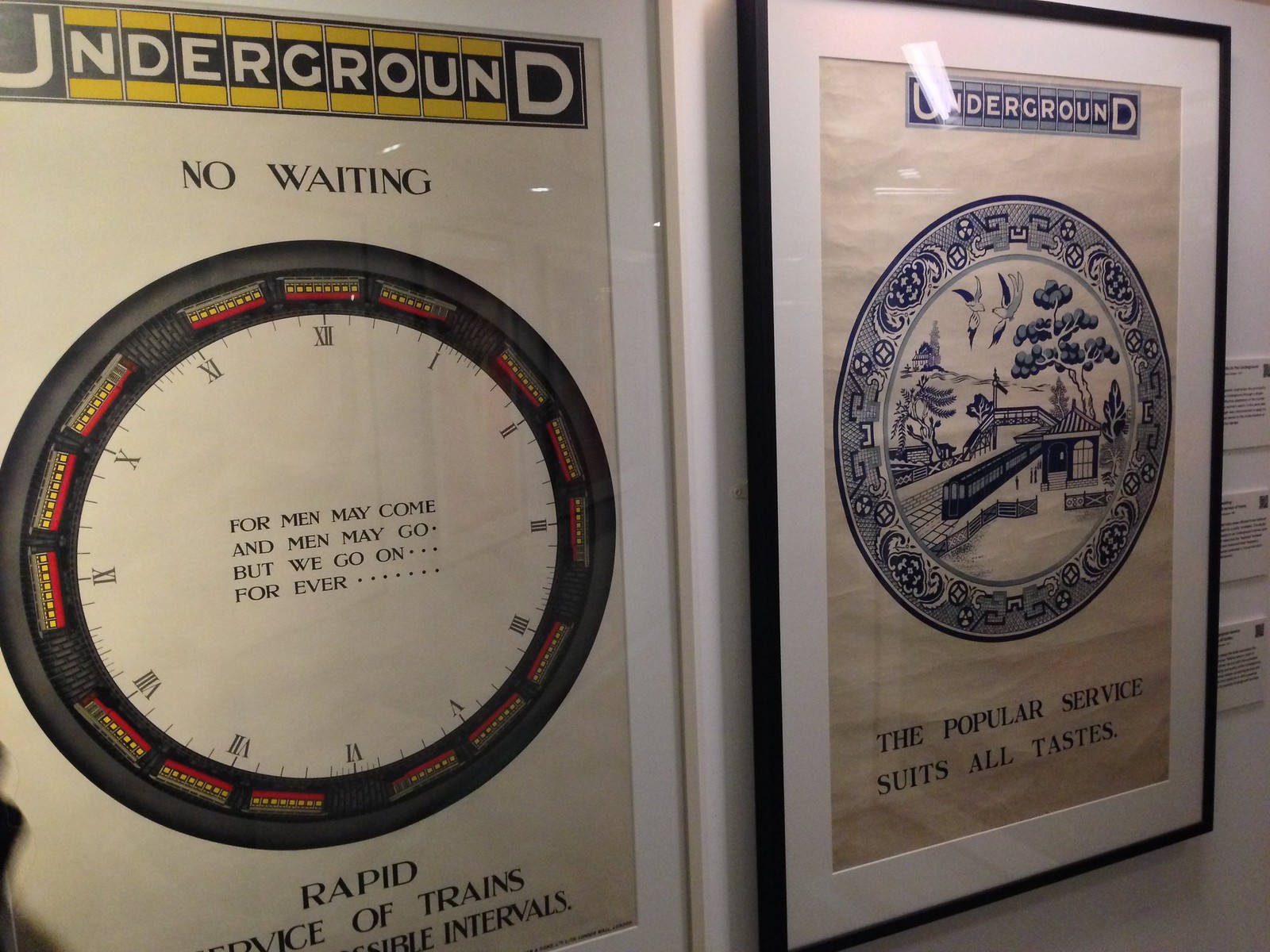The image depicts two framed posters hanging on a wall, each promoting the concept of underground train services. The poster on the left is encased in a white frame with a white background. It prominently features the word "UNDERGROUND" in large black letters at the top, followed by "NO WAITING" beneath it. Dominating the center is an abstract clock face with Roman numerals, accented in black, yellow, and red. Inside the clock face is the phrase “FOR MEN MAY COME AND MEN MAY GO, BUT WE GO ON FOREVER,” signifying the perpetual nature of the service. Below the clock, partially cut off but visible, are the words "RAPID SERVICE OF TRAINS."

The poster on the right, housed in a black frame, features a white background with blue elements. At the top, "UNDERGROUND" is displayed in white letters against a blue backdrop. Central to this poster is a circular image depicting a train moving through a scenic background, complete with birds and trees. Beneath this visual, the text reads "THE POPULAR SERVICE SUITS ALL TASTES" in blue lettering. Both posters, rich in detail and color, appear to serve as vintage advertisements for a reliable and efficient underground train service.